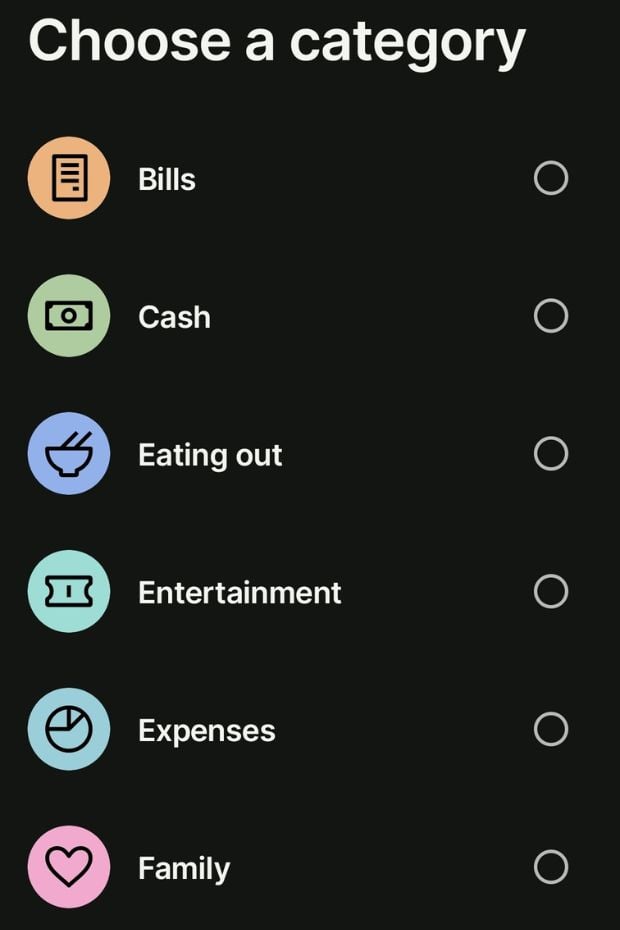This image captures the screen of a smartphone displaying a selection menu against a black background. At the top, in white text, it reads "Choose a category." Below this header, there are three distinct columns. 

The first column contains six colored icons arranged vertically:
1. An orange icon labeled "Bills."
2. A green icon resembling a dollar bill labeled "Cash."
3. A blue icon depicting a bowl with silverware labeled "Eating Out."
4. An icon resembling a clapperboard labeled "Entertainment."
5. An icon of a pie chart labeled "Expenses."
6. A pink heart icon labeled "Family."

The second column contains the text labels that correspond to each of these icons.

The third column features interactive black circles outlined in white, which can be clicked to select a category. As observed, none of these circles have been selected, as indicated by the absence of checkmarks or dots.